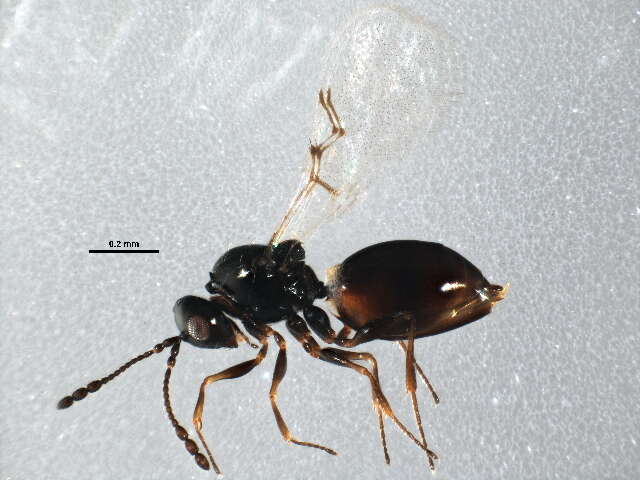This detailed image captures a close-up of a bug, likely an ant based on the majority of descriptions, though there's a suggestion it could be another type of insect like a bee. The insect is positioned centrally in the lower part of the image, lying on its side against a light gray background speckled with white. To the left of the insect, there is a horizontal line labeled "0.2 mm," indicating a measurement scale.

The insect's head, slightly tilted downward and facing left, is black with an eye reminiscent of a fly's compound eye. Extending from its head are two long antennae; one stretches downward to the left, while the other curls back to the right. Behind the head, the insect has a round black thorax, followed by a larger dark brown abdomen featuring a notable protrusion with small yellow extensions. The insect has multiple legs; one extends upward in the image, while several others, likely from the right side, project downward due to the perspective of the photograph.

Given the precision and the presence of the measurement scale, the image appears to be part of a scientific study or educational material, possibly aimed at examining the insect's anatomy and physiology.